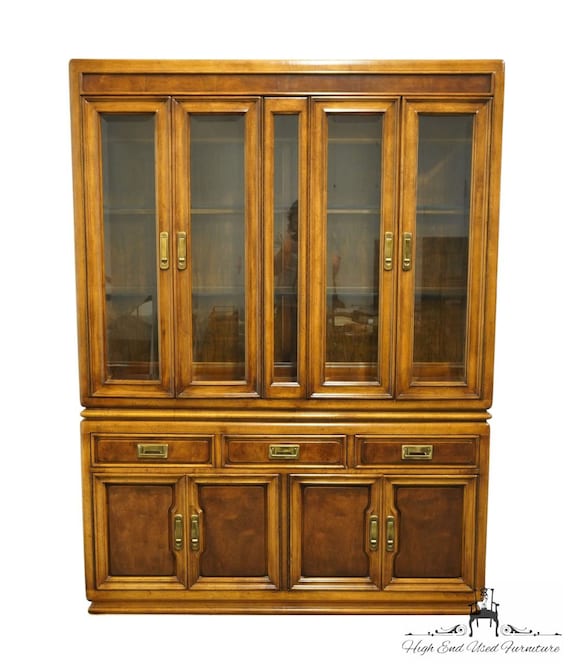The photograph captures a vintage wooden hutch, showcasing a blend of intricate design and functional storage. The hutch, stained with a mix of dark and light spots, echoes a sense of antiquity. Its top section features two sets of large glass-paneled double doors, each adorned with gold handles. Through the clear glass, you can spot two shelves within each section. Beneath these glass doors, there are three horizontal drawers, also equipped with gold handles. Situated below these drawers are two smaller, more compact cabinets, each with double doors and matching gold handles. The furniture piece is devoid of any contents, providing a clear view of its internal structure. Notably, in the bottom right corner of the hutch, there's a logo depicting an ornate wooden chair accompanied by the inscription 'High-End Used Furniture' in an elegant script font.